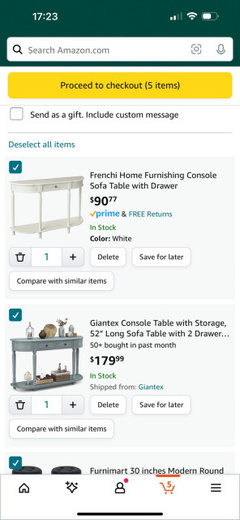In this detailed image, we see a screenshot of an iPhone interface captured at 5:23 PM, as indicated by the time displayed in the top left corner. In the top right corner, there are icons representing the network signal strength, Wi-Fi connectivity, and the current battery level.

Central to the image is a search field and a series of text elements related to an online shopping cart or checkout screen. The text reads "Proceed to checkout" and mentions "Five items." Additionally, there are options like "Send us gifts" and "Include custom message."

The products listed in the cart are: 
1. **Frenchie Home Furnishings Console** - A sofa table with a drawer, priced at $19.77.
2. **Glantez Console Table with Storage** - A 52-inch long sofa table featuring two drawers, with a price tag of $179.99.

Towards the bottom of the screenshot, the iPhone home button is visible along with icons for the shopping cart and the menu, indicating typical navigation options found in an e-commerce application.